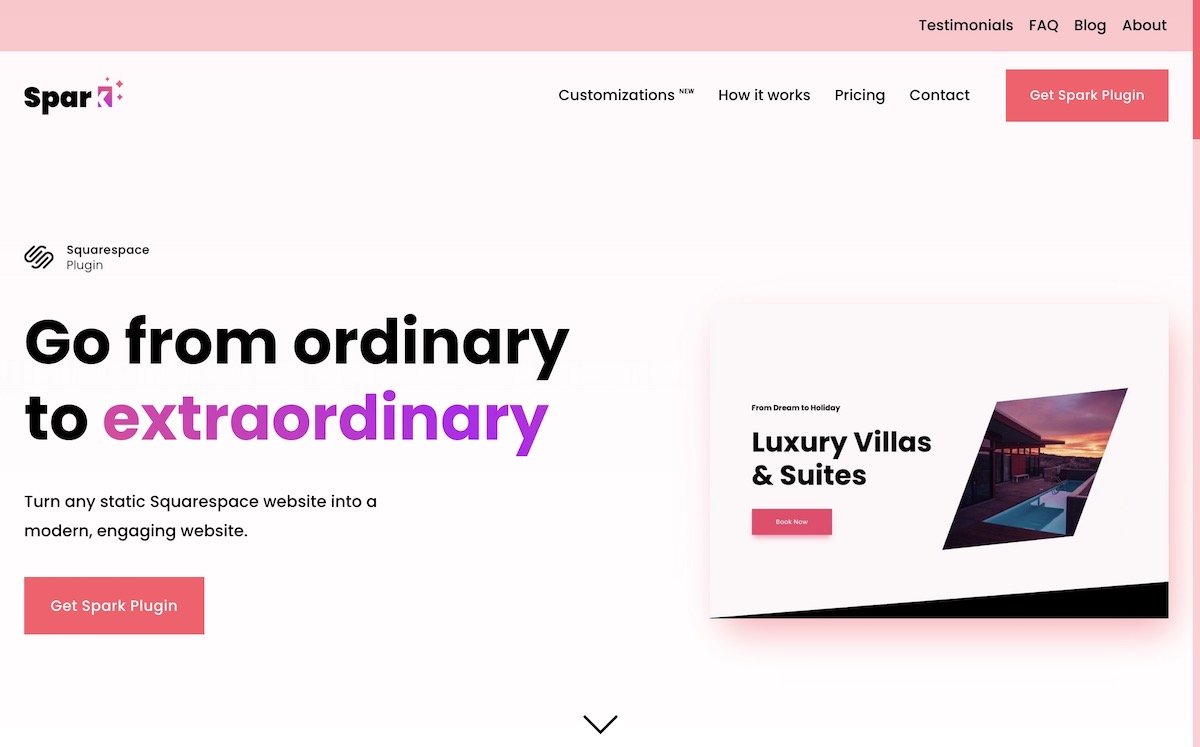This is a detailed caption for the image of the Spar website:

The Spar company website features a modern and engaging design. At the top, a prominent pink strip offers easy navigation with four options: Testimonials, Frequently Asked Questions, Blog, and About. Below this, the company’s name, 'Spar,' is displayed alongside their distinctive logo—a pink square featuring an angled white line that rises and curves to the right, surrounded by three dots on the right side.

Directly beneath the logo, Spar's tagline catches the eye: "Go from ordinary to extraordinary." The words "Go from ordinary to" are in large black letters, while "extraordinary" stands out in even larger pink letters. Further down in smaller print, another tagline reads, "Turn any static Squarespace website into a modern engaging website."

The website also highlights various sections such as Customizations, How It Works, Pricing, and Contact, along with a prominent call-to-action button labeled "Get Spark Plugin" in a pink-colored box with white lettering.

On the right side of the page, there's an image of a picturesque villa at sundown, featuring a luxurious pool in the foreground. Overlaid on this image is the caption "Luxury Villas and Suites" in black text. Below this, another pink box contains small text that is difficult to read. 

Overall, the sleek layout and vibrant color scheme of Spar’s website are designed to captivate and convert visitors by showcasing the transformative power of their Spark plugin for Squarespace sites.